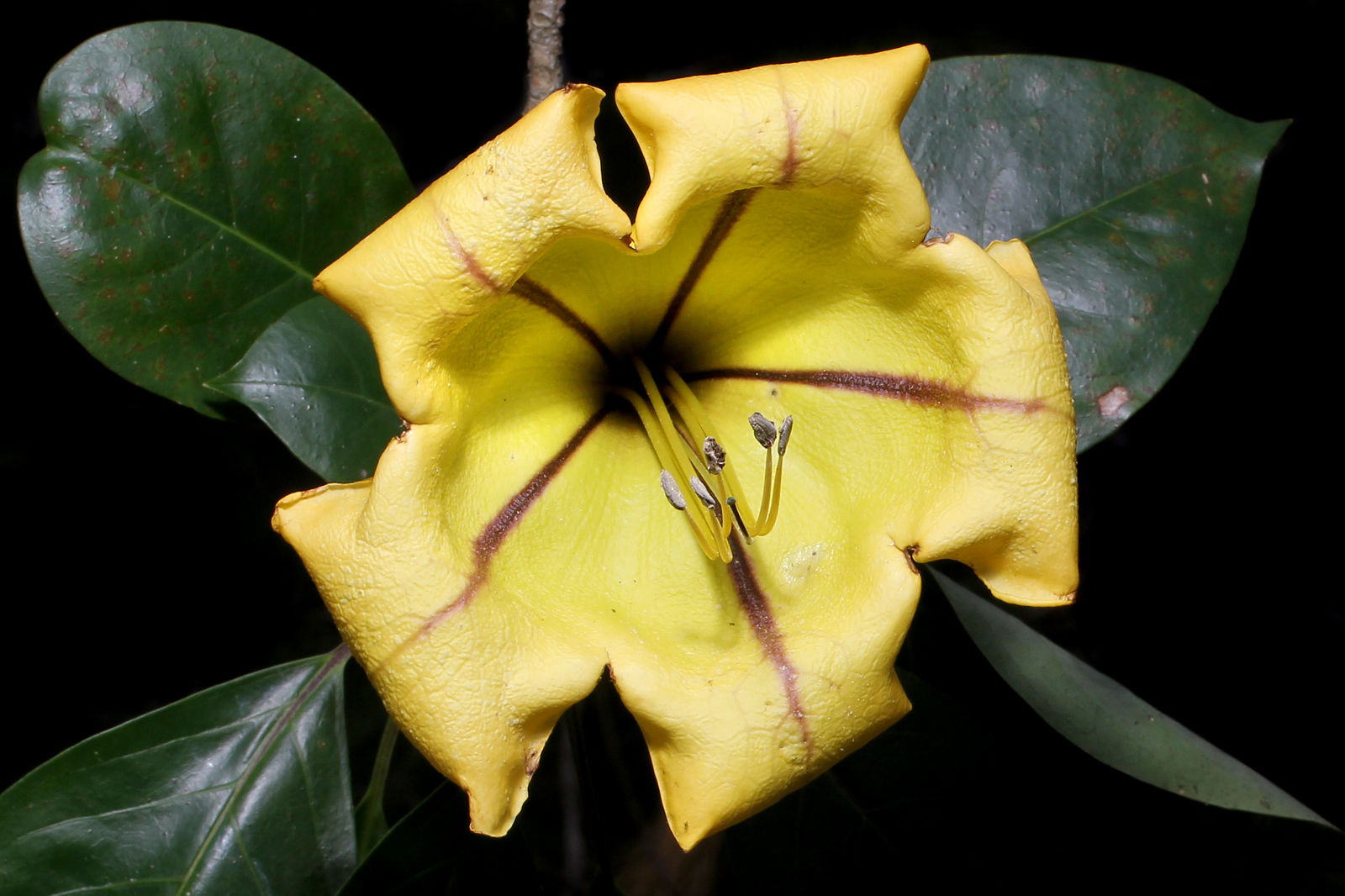In this detailed close-up photograph, a single yellow flower takes the center stage against a pure black background, giving it a dramatic and professional appearance. The flower, possibly in a state of blooming or wilting, exhibits five petals that curve backward, resembling an inside-out effect. Each petal is adorned with a distinct purple line running through the middle, adding to its intricate beauty. The petals range from a darker yellow at the center to a nearly white faded yellow at the tips. Emerging from the flower's core are yellow filaments, each capped with a tiny white-brownish ball at the tip.

Surrounding the flower are at least five thick, dark green leaves that enhance the vibrant contrast between the flower and its background. Notably, the leaf on the bottom right displays a small white spot indicating the onset of deterioration, while a nearby leaf curls slightly to the left. A bit of the flower's small stem is also visible peeking from the top of the image, completing this detailed visual narrative.